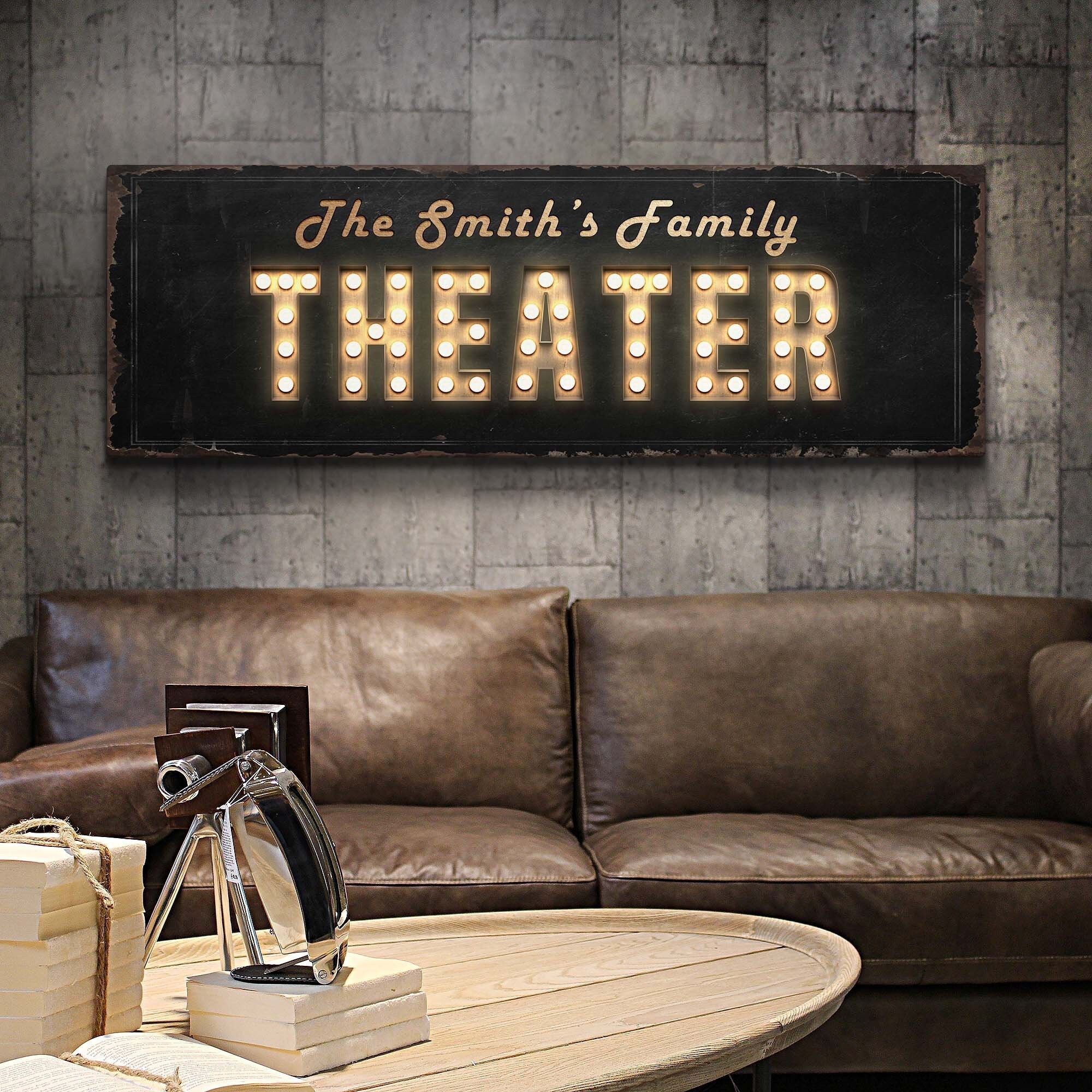In the image, a cozy theater room is depicted, dominated by a large, plush brown leather couch with two substantial rectangular seats and back cushions. The couch also features an armrest for added comfort. Positioned prominently on the gray, slate-like wall behind the couch is a black poster with chipping paint along the edges, which reads "The Smiths Family Theater" in glowing gold, cursive letters, reminiscent of classic movie theater signage.

In front of the couch stands a circular, light tan-brown oak table that holds several items. A striking vintage camera with a mix of brown and chrome detailing is set up on the table, directed towards a stack of seven or eight books that are either white or tan, some bound with twine. Next to these items, there is a chrome device, partially black, which may resemble a clock or a large watch head. The room's warm, inviting atmosphere is highlighted by the thoughtful arrangement of furniture and decor, making it an ideal space for family entertainment and relaxation.